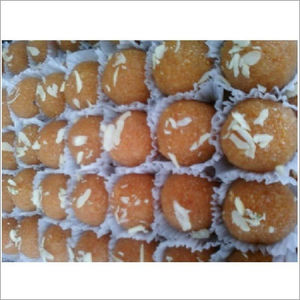The image is an overhead shot displaying several rows of uniform, spherical pastries nestled in white paper liners, akin to those used for cupcakes or chocolates. Each pastry is beige and appears to have a dense, cake-like texture, reminiscent of donut holes. The surface of these pastries glistens slightly, suggesting a coating of fine sugar crystals. Sparsely sprinkled on top of each pastry is a hint of white coconut flakes, adding texture without overwhelming the overall appearance. The pastries are tightly arranged, with the visible portion of the image showing about 18 to 20 pastries, although the rows seem to extend beyond the frame. The photograph is bordered by a white band on the top and bottom, emphasizing the close-up perspective and the neat alignment of the treats.